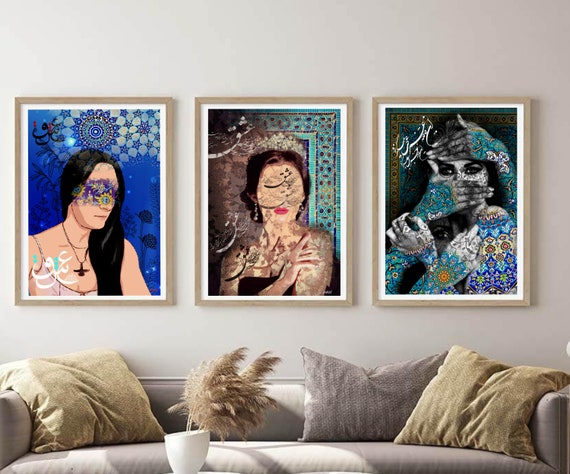The staged living room features a beige or gray wall adorned with three vibrant and colorful paintings, each depicting a woman. The leftmost painting predominantly utilizes blue shades, with kaleidoscope shapes and floral patterns covering the woman's face, obscuring her eyes. Her long black hair cascades down past her breasts, and she is adorned with a brown or black necklace and a pink dress. The center painting features a woman with short hair, wearing a beige crown and a brown dress. Her eyes are similarly obscured, resembling Picasso's style, but her reddish-pink lips are visible. The background transitions from a brown left side to an intricate, rug-like pattern on the right, composed of brown, cyan, and dark blue dots on a greenish-blue color. The rightmost painting shows a woman whose forehead and mouth are covered by hands decorated with cyan kaleidoscope shapes. Her face is gray with visible eyes, and her black hair flows around the gray, unpainted parts of the hands. The shoulder in the painting is adorned with cyan and blue floral and kaleidoscope-like objects. Below the paintings, a gray couch is positioned with beige or tan pillows on either end, a gray pillow, and a white vase on a table holding tan or beige plants.